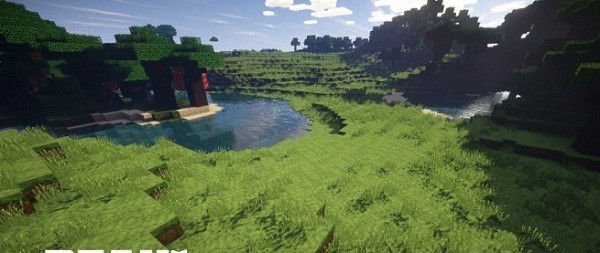This image, resembling a scene from the video game Minecraft, depicts an outdoor landscape with vivid detail. The sky is a deep blue adorned with white clouds in the distance. Green grass, arranged in terraced levels, dominates the foreground, creating an impression of ascending stairs. A lagoon, featuring pristine blue water, lies in the center of the image; it includes a small island with trees on it. On the right side, there is another water body partially obscured by a shadow. In addition to natural elements, a burgundy structure with block-like features—typical of Minecraft construction—stands on a sandy bank beyond the central lagoon. The background is graced with hills topped with both realistic and pixelated trees, enhancing the picturesque vista.